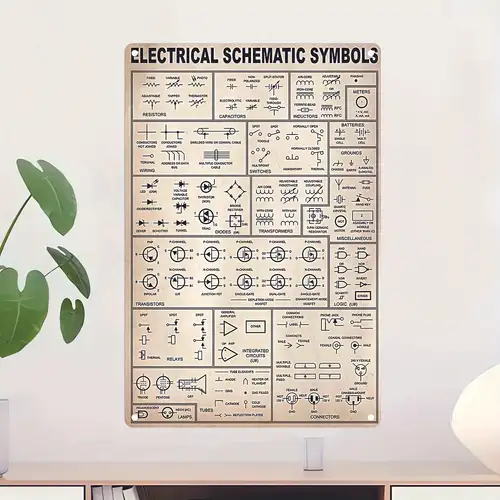The photograph showcases a rectangular metal sign mounted on a plain white wall, prominently displaying "Electrical Schematic Symbols" at the top. The sign is covered with an array of symbols, each accompanied by explanatory text, but the small size and slight blurriness of the image make the words unreadable. The symbols, representing various electrical components and functions one might encounter in a breaker box or technical manual, are intricately detailed.

Beneath the sign, a shelf with visible books supports a neatly arranged scene. To the left of the shelf, a potted plant with sprawling green leaves adds a touch of greenery, partially extending into the frame. Positioned towards the bottom right of the shelf, a round, white object is discernible, though its specific function remains unclear. The overall atmosphere is one of organized technical reference juxtaposed with a hint of natural decor, all captured in a compact, detailed frame.